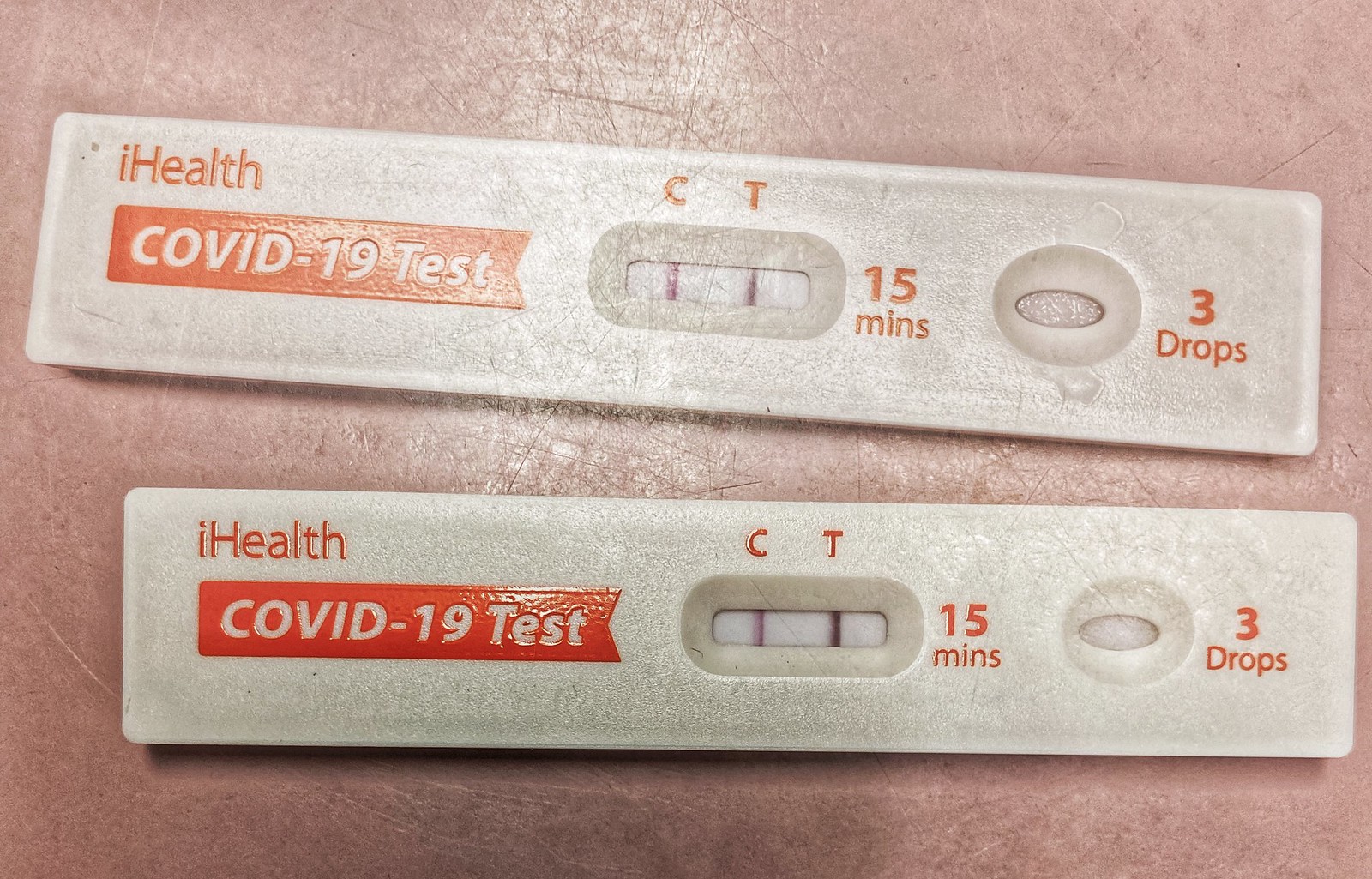This is a detailed photograph of two COVID-19 rapid test kits positioned on a heavily scratched, pink flat surface. Both test kits are white and bear the label "Eye Health" in orange lettering at the top left corner. Below this, within an orange flag-like shape, is the text "COVID-19 Test." 

Each test features a small window in the middle, bordered by gray, displaying the letters "C" and "T." Both tests show a reddish-purple line under "C" and another under "T," indicating positive results. Adjacent to the window, "15 MINS" is printed, signifying the recommended time for result reading. Below the window is an oval-shaped opening labeled "3 drops" in orange, indicating where samples are to be placed.

The two tests are arranged with the top one slightly crooked and the bottom one perfectly aligned with the surface. Both tests appear worn, with visible scratches. Additionally, the upper test shows signs of dried liquid around the sample drop area, further indicating use.